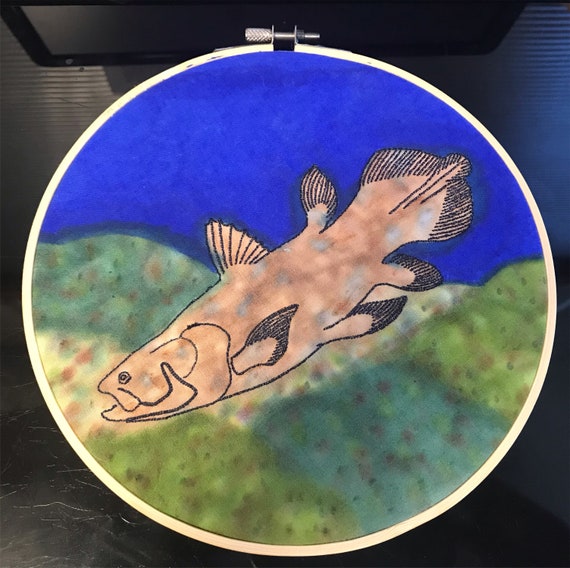This is a detailed close-up image of a completed needlepoint piece held taut by a light-colored wooden embroidery hoop with a silver clasp at the top. The needlepoint depicts a large fish spanning the width of the hoop. The fish, possibly a catfish, is intricately stitched in mottled rusty brown with black stitching details, and adorned with blue, pink, and whitish dots. It swims with its mouth open towards the left side of the image. Above the fish, the fabric resembles deep blue water, transitioning into a greenish-brown background below, hinting at the underwater riverbed. The whole setup is positioned on a black table and leans against a white wall, with part of a television screen with a black border slightly visible at the top of the photo.